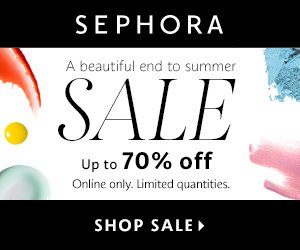"Sephora Sale Promotion: 

The graphic features a striking design with the top and bottom halves in sleek black, while the middle section is highlighted in white. At the top, 'Sephora' is prominently displayed in white text. Below, the phrase 'Shop Sale' is also written in white, anchoring the design. In the center, bold and emphatic black text announces a sale with discounts up to 70% off, exclusively available online. The phrase 'Limited quantities' is written below in a smaller, yet clear black font. Adding a vibrant touch, various shades of makeup are artistically smeared across the graphic: bright blue powder, rich red lipstick, a dot of yellow paint, soothing green lotion, and a dash of pink blush. The phrase 'A beautiful end to the summer' is elegantly written in grey, encapsulating the essence of the sale. The word 'Sale' is especially emphasized in large, bold letters, making it stand out. The entire graphic is carefully composed within a perfectly balanced small square, with each line featuring a distinct font to enhance readability and visual interest."